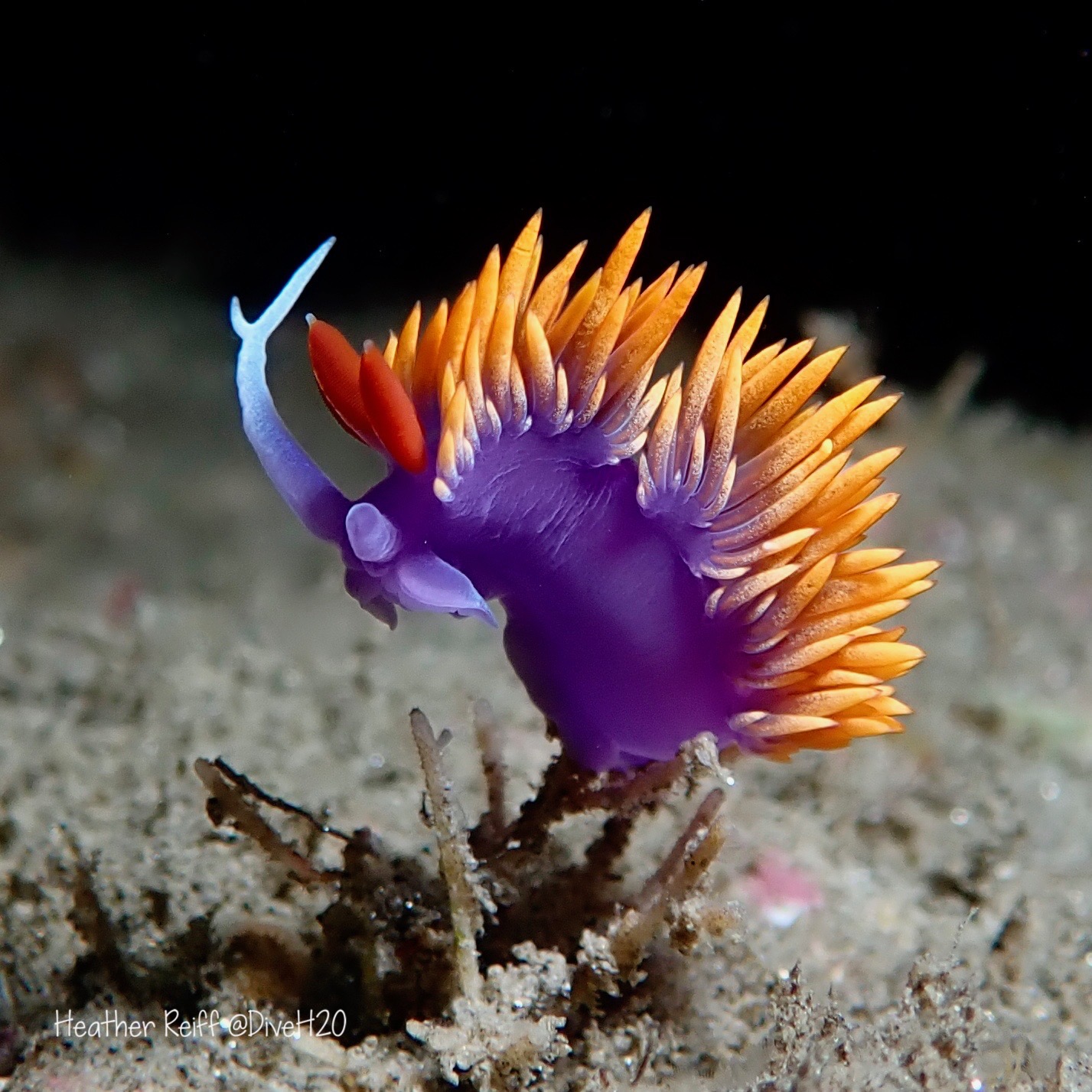The image features a close-up photograph of a vibrant underwater scene, showcasing a curious marine organism that resembles a young sea anemone. The background is pitch black, accentuating the organism at the center of a wide vertical frame. The ground is a sandy brown, dotted with small stones and sticks.

In the middle of the frame, there are two brown sticks rising from the sand, supporting a prominent purple centerpiece. This structure features a deep purple hue, leaning to the left, with a distinct appendage protruding horizontally before bending upward. At the top of this appendage, it splits into two thin rectangular shapes. Surrounding the purple body, the back side is adorned with a dense array of orange, dark orange, and yellow cylindrical spines topped with pointed tips, creating a forest-like texture.

Notably, two of the spines on the left are red, complemented by a limb transitioning from purple to light blue. This organism vividly comes to life, bearing a striking resemblance to a blossoming sea anemone. At the bottom left corner of the image, there is white text that reads "Heather Reif, R-E-I-F-F, at dive H20."